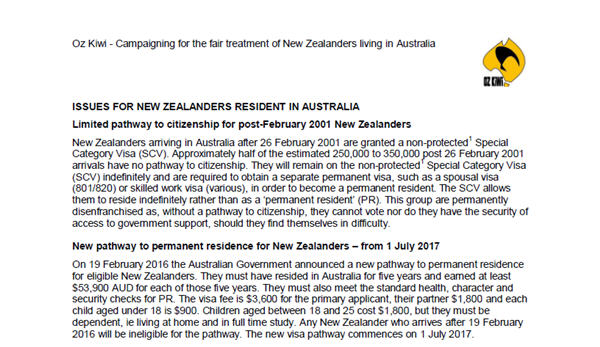This image features a screenshot set against a white background, displaying important information in dark grey text at the top. The text reads: "A'az Kiwi campaigning for the fair treatment of New Zealanders living in Australia." To the right of this text, there is a yellow logo with a black swirl in the center, adding a touch of visual interest. 

Below this, the background changes to a light grey, providing the backdrop for more detailed information. The bold heading states: "Issues for New Zealanders residents in Australia." Subsequently, the text explains the specific issue: "Limited pathway to citizenship for post-February 2001 New Zealanders." It further elaborates that New Zealanders who arrived in Australia after 26 February 2001 are granted a non-protected Special Category Visa. Shockingly, approximately half of the estimated 250,000 to 350,000 post-26 February 2001 arrivals have no pathway to citizenship, leaving them on the non-protected Special Category Visa indefinitely.

The next section, introduced with bold text, outlines a new development: "New pathway to permanent residence for New Zealanders." This segment presumably provides hope and potential solutions for those affected by the previous restrictive policies, aiming to address the citizenship pathway issues faced by New Zealanders living in Australia.